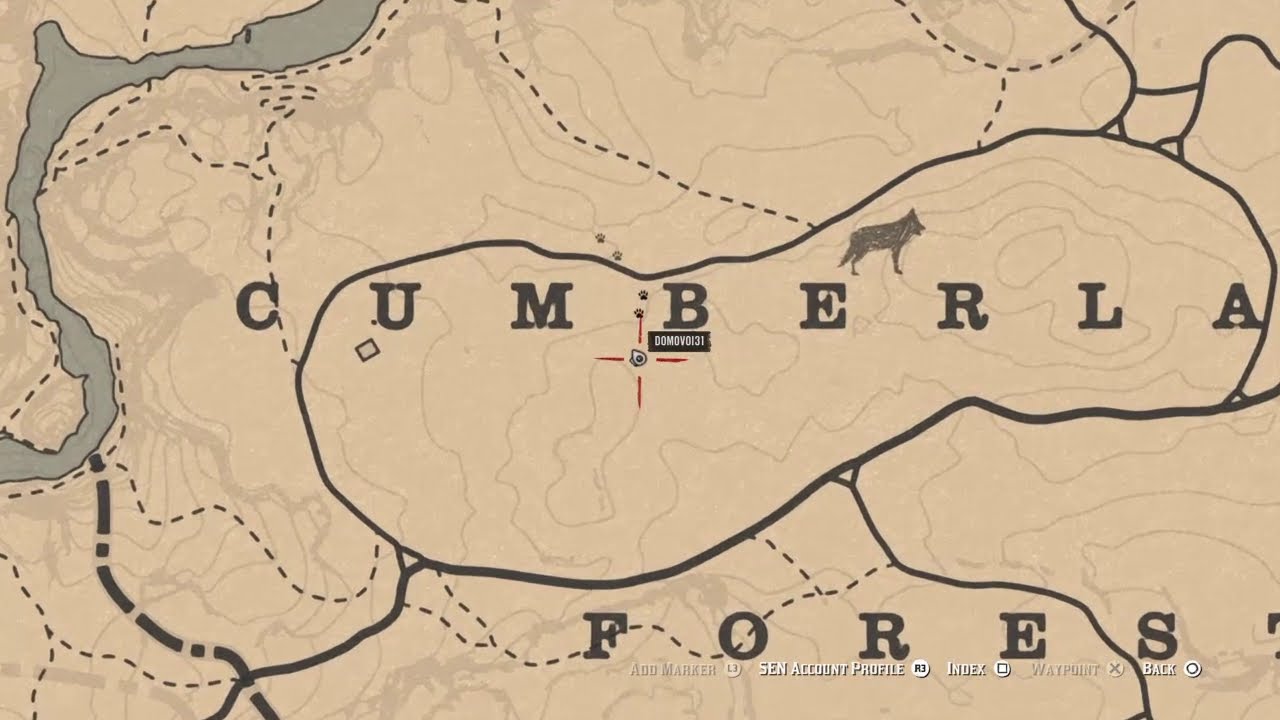The image presents a detailed section of a cartographic map with a predominant beige background and light tan shading, characteristic of topographic illustrations. Central to this map is the region labeled "Cumberla," with the accompanying word "Forest," albeit with the T extending off the right-hand side of the page. The lettering is in bold black, visibly spaced out. Above the text "Cumberla," there's a sketched grey pencil outline of a wolf, depicted from its right side. The map features multiple drawn elements, including dark black roads, dotted and solid lines, and terrain indicators. Towards the top left to the midway of the left-hand side, a river is illustrated in blue. The terrain lines depict mountain ranges, primarily on the left and bottom sections, in a beige tone. The entire layout appears to include elements like geometric shapes and dotted line paths indicative of varied terrains and possibly routes within the map.